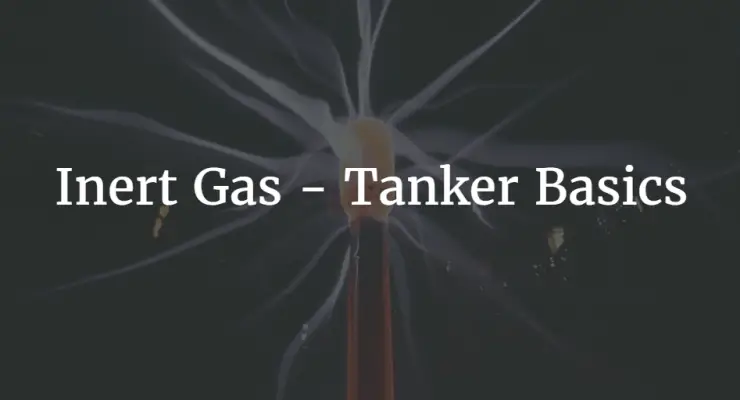The image is a horizontal rectangle poster with the white text "INERT GAS - TANKER BASICS" prominently displayed at the forefront. The background, hazy and darkened, features a faded, detailed depiction of a lit match. The match's bottom part is reddish and transitions to a golden glow at the top. From the matchhead emanates wispy, white-gray smoke, which curls and diffuses against the dark blue or black backdrop. The smoke appears almost ethereal, akin to electric threads or long, stringy tendrils. On the right edge of the image, a broken-off fragment or piece seems slightly out of place, adding an enigmatic touch to the composition. The overall visual is subdued, emphasizing the crucial informational text while maintaining a mysterious, smoky ambiance.